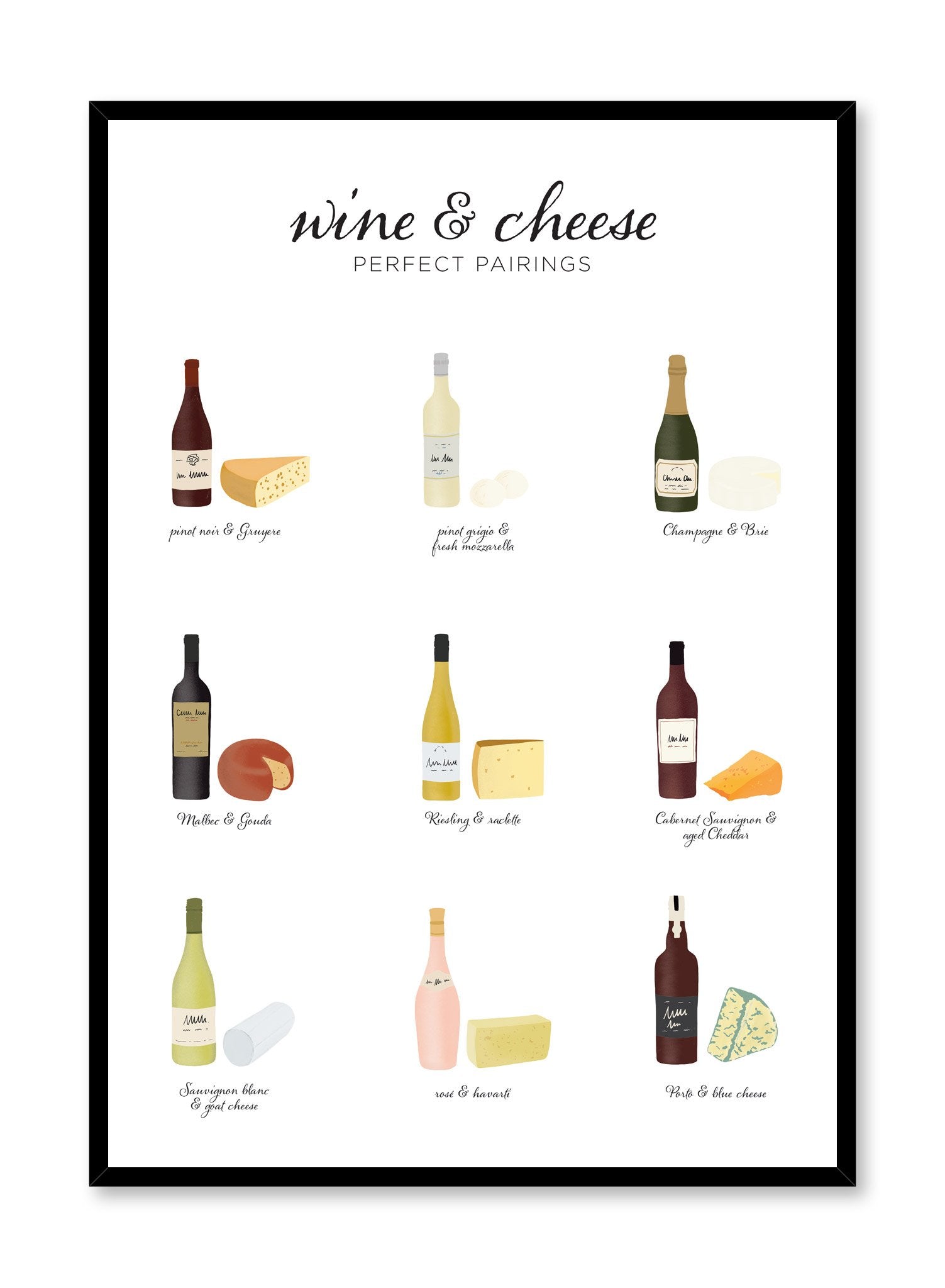This vibrant and detailed poster, titled "Wine and Cheese: Perfect Pairings," features nine delightful wine and cheese pairings arranged in three rows and three columns. Encased in a sleek black frame, the poster's bright white background makes the colorful, yet basic caricatures of the wines and cheeses pop. The caption at the top reads "Wine and Cheese" in an elegant, easy-to-read cursive font, followed by "Perfect Pairings." Each wine and cheese pairing is artfully illustrated, providing a charming visual guide. The pairings include Pinot Noir with Gruyère, Pinot Grigio with fresh mozzarella, Champagne with Brie, Malbec with Gouda, Riesling with Raclette, Cabernet Sauvignon with aged cheddar, Sauvignon Blanc with goat cheese, Rosé with Havarti, and Port with blue cheese. This aesthetically pleasing and informative print would make an ideal accent in any culinary space, celebrating the classic harmony of wine and cheese.